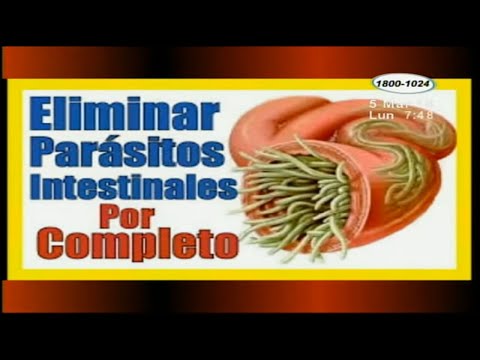The image features an advertisement with a black background, focusing on the human anatomy, specifically the intestines. The central element is a digital rendering of a coiled, pinkish-red depiction of intestines, featuring green, worm-like parasites. The text on the left side of the image is written in Spanish and includes phrases like "Eliminar Parasitos Intestinales Por Completo," which suggests it is promoting a product or service for the complete removal of intestinal parasites. The text is blue and red on a white background, with a red and yellow outline framing the entire image. The background of the intestines is darker red, making the details stand out prominently. The overall visual presentation is striking with its bold colors and vivid anatomical illustration.